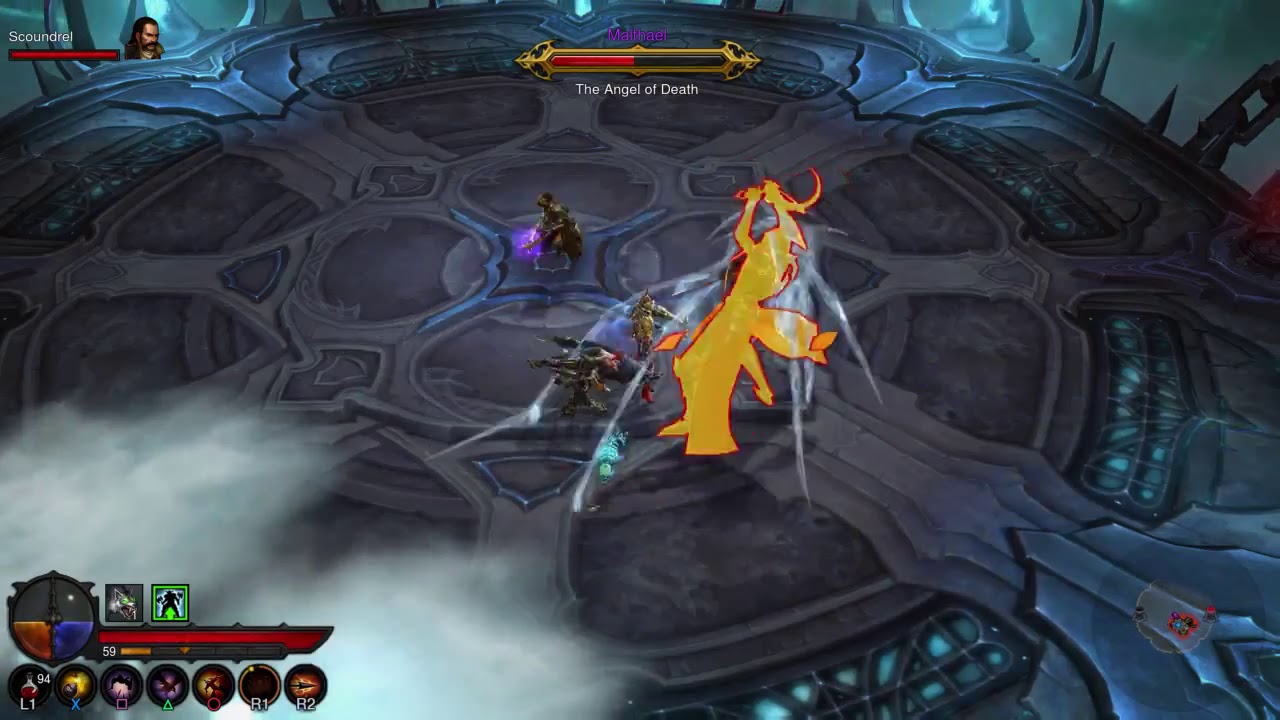This screenshot captures an intense moment within a fantasy-themed video game, possibly League of Legends. The scene is set on a large, grey, circular platform elevated in the air, connected by multiple bridges. At the center of the action, three to four characters wielding swords and other weapons are engaged in combat with a massive yellow and red-bordered figure identified as the Angel of Death. The Angel of Death's partially depleted health bar is prominently displayed at the top center of the screen. In the upper left corner, there is a character named Scoundrel, whose fully filled health bar and face icon are visible. The bottom left corner features various icons, health bars, and actionable buttons integral to gameplay. The overall scene exudes a dynamic and immersive fantasy combat atmosphere.